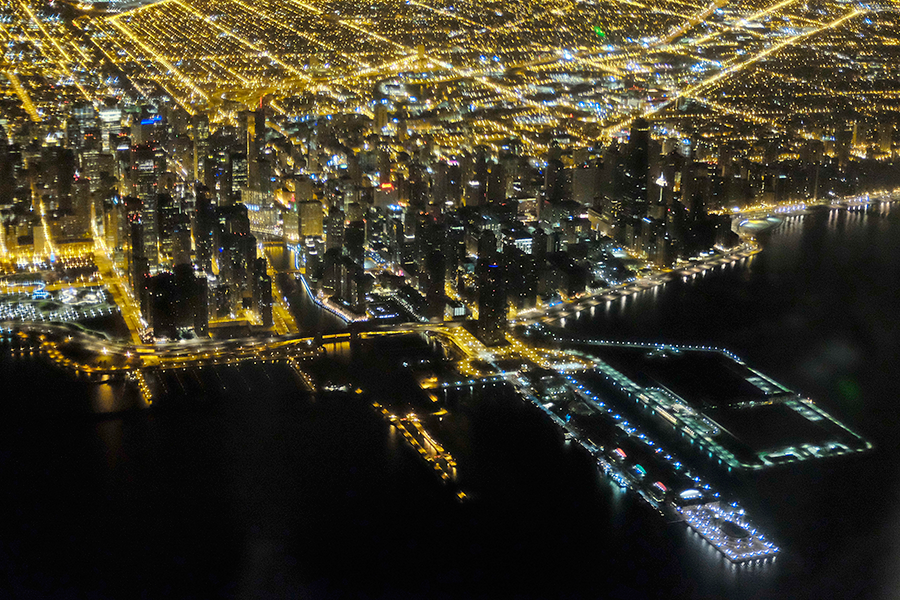This aerial nighttime photograph captures the expansive downtown of a bustling city, showcasing a stunning interplay of light and architecture. The bottom third of the frame features a dark, pitch-black river, adorned with a variety of illuminated piers. On the left, a small marina glows with orange lights on either side, while to its right, a longer pier extends further into the water, also adorned with orange lights. Further to the right, an even longer pier, illuminated by blue and yellow lights, reaches into the river. Adjacent to this is a medium-sized marina with distinctive greenish lights.

The prominent skyline behind the river is dominated by numerous tall, mostly dark gray skyscrapers, punctuated at intervals by vibrant yellow, red, and white lights that highlight their structures. In the distance, a vast grid of roads is visible, lit by orange streetlights, outlining the city's intricate layout with smaller buildings nestled in between the illuminated streets. The lights scattered throughout the scene resemble speckles of gold glitter, accentuating the vibrancy of this large, densely populated city.